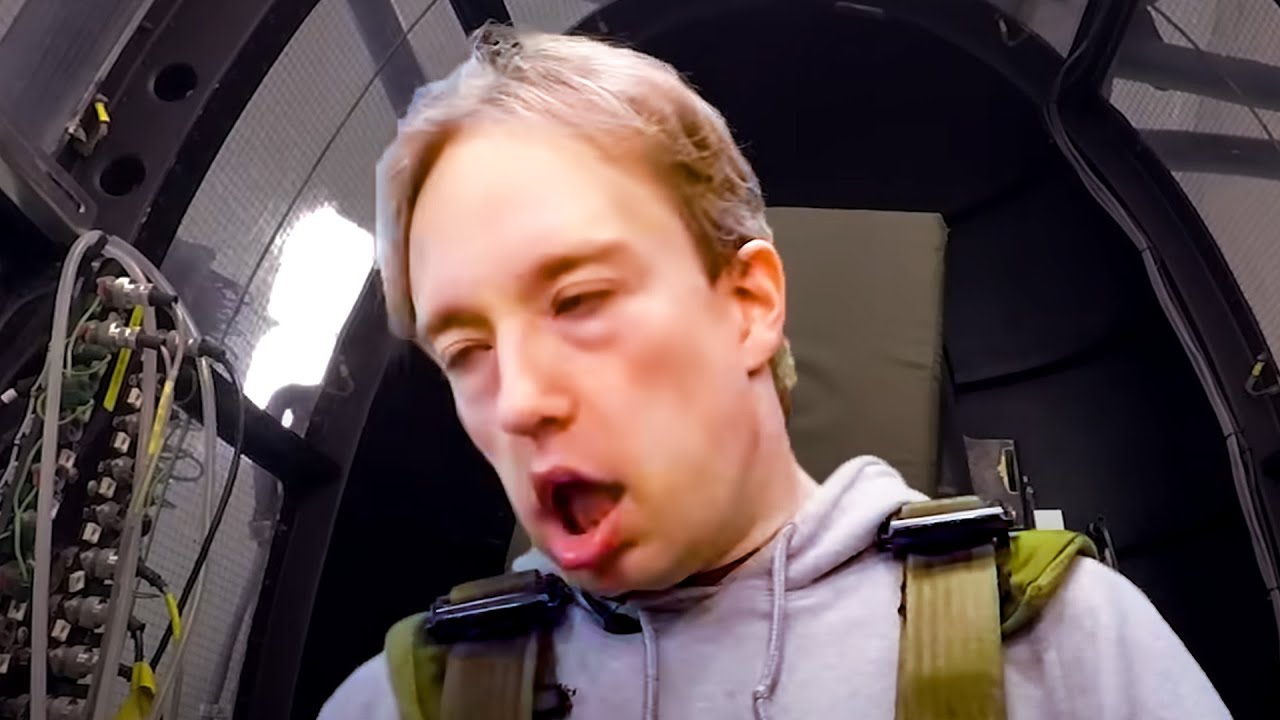The image depicts a somewhat disfigured-looking man in a gray hoodie who appears to be experiencing intense g-forces or motion, likely on some sort of aircraft, rollercoaster, or g-force trainer. His face is heavily distorted, with his mouth agape and his eyes rolling back, giving an impression that he might be about to throw up or has just passed out. The short gray hair of the man is blown back, adding to the sense of high-speed motion. He is strapped into a seat with green straps over his shoulders, which is part of an ovular or egg-shaped chamber. This machine is filled with cables and plugs next to him, featuring gray and yellow wires, indicating a high-tech or mechanical setting. The black oval behind him and the gray roof surrounding it suggests he is enclosed within this device, possibly under some physical testing.